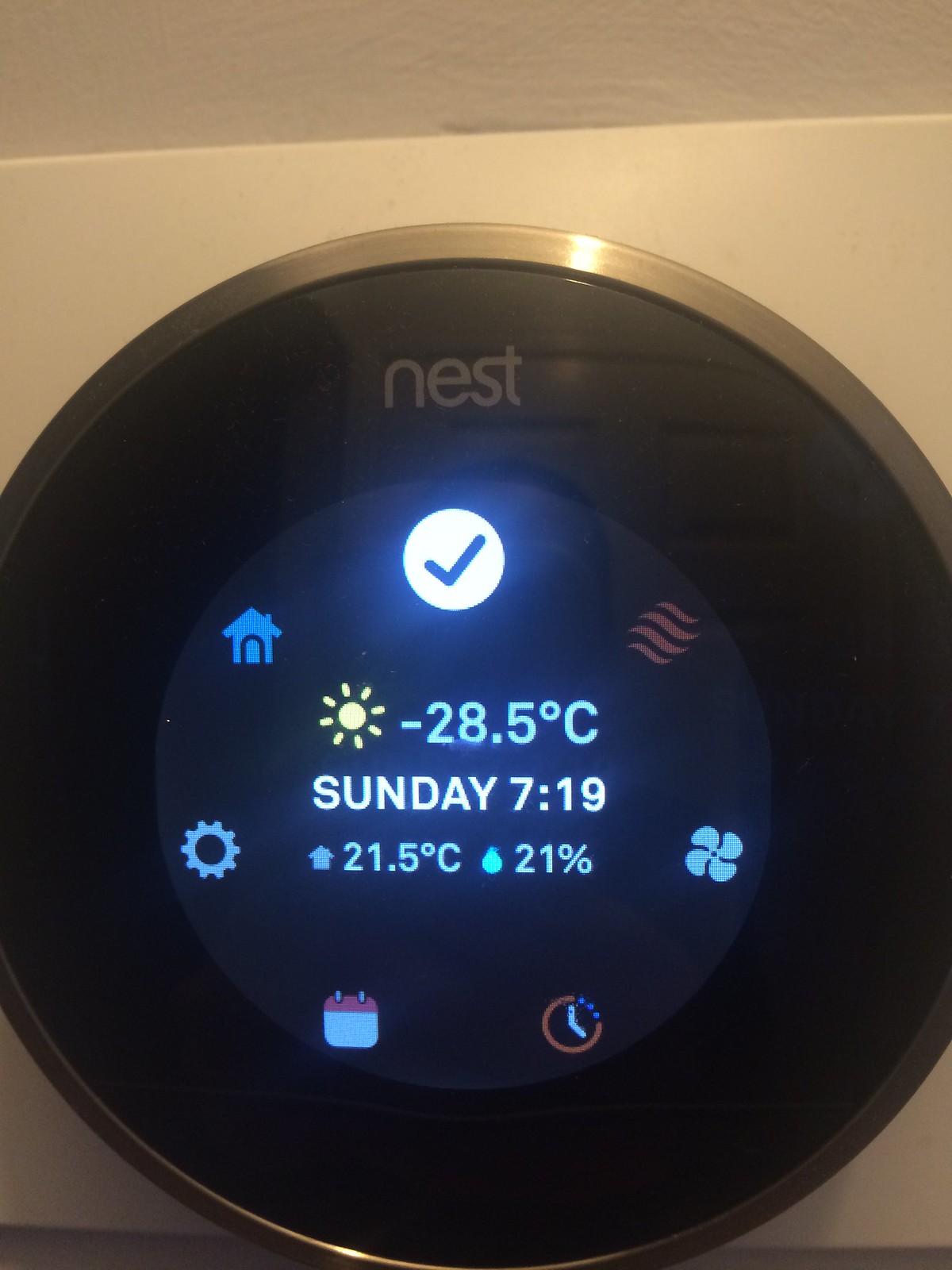The close-up image depicts a Nest thermostat mounted on a white wall. The device features a gold ring encircling its black face, which prominently displays a host of details. At the top, the brand name “Nest” is shown in white lettering. 

In the center of the display, various icons and information are visible. On the bottom left, there is a gear icon indicating settings. Adjacent to it is a house icon, alongside a blue check mark symbolizing confirmation or correct status. The right side includes a heat symbol and a fan icon with a timer underneath. 

The screen displays the current temperature of -28.5°C along with the current date and time: Sunday, 7:18:19. The thermostat is set to an in-house temperature of 21.5°C with a humidity level of 21%. 

Overall, this high-tech device is accentuated by its minimalistic and sleek design, with a clear and informative interface.